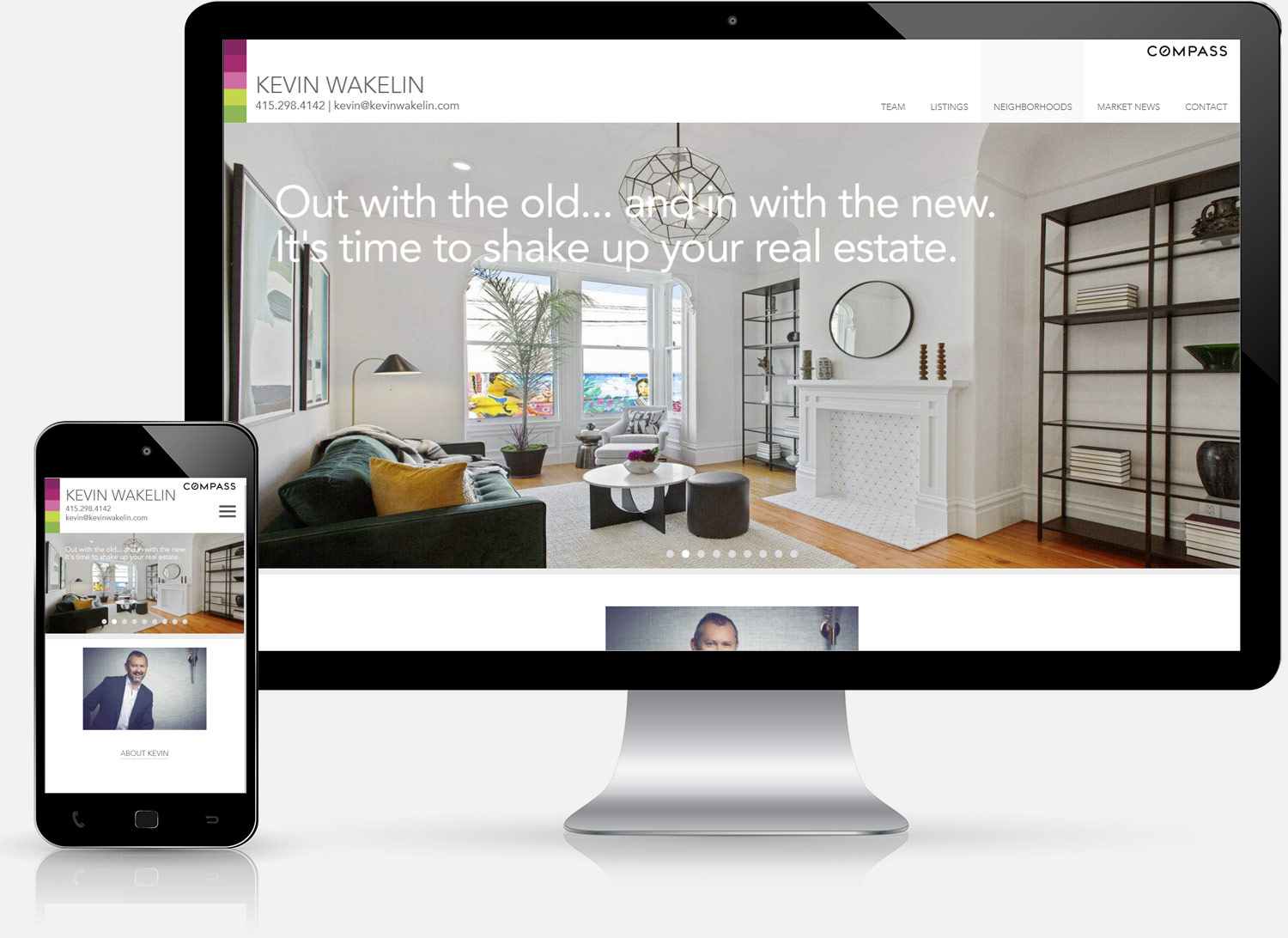The image showcases an Apple computer monitor displaying a real estate advertisement. Prominently featured in the top right corner is the word "Compass" set against a white bar that spans the width of the screen. Below this, the name "Kevin Wakelin" is displayed along with a contact phone number and email address. Taking up the central portion of the screen is a pristine living room with white walls. The room is impeccably organized, featuring a sleek black bookcase on either side, constructed of thin wire and metal. 

In the center of the living room stands an all-white fireplace adorned with a round mirror. To the left, a dark-colored couch is positioned, accompanied by framed pictures overhead. A close-up image of a man's face, showing only from his nose upward, appears in a square at the bottom of the screen, with a small object visible to the right of his face. The caption on the screen reads: "Out with the old and in with the new. It's time to shake up your real estate."

In the lower left corner of the photograph, a smartphone is visible. The phone shows the same real estate image, but additionally includes the full view of the man's face and upper body, set against a white background.